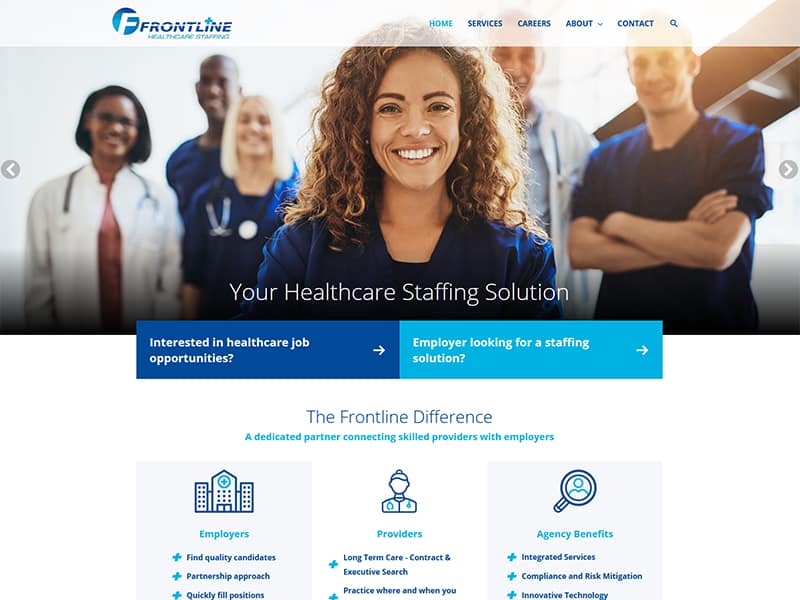**Frontline Healthcare Staffing Web Page Overview**

At the top of the web page, a white banner displays the text "Frontline Healthcare Staffing" prominently. Above this banner, the navigation options include 'Home' (highlighted in light blue) followed by 'Services', 'Careers', 'About', 'Contact', and a search icon, all in dark blue.

The central image on the page features a group of diverse medical professionals. At the forefront is a Hispanic woman with curly, brownish hair, beaming a wide smile and dressed in dark blue scrubs. Surrounding her are other slightly blurry healthcare workers, showcasing diversity in the team. To her left stands an African-American woman with short black hair, clad in a doctor's coat and stethoscope. Beside her is an African-American man with a bald head, wearing a dark blue T-shirt. In front of him is a white woman with shoulder-length blonde hair, also wearing scrubs and a stethoscope. To the right, partially visible, is a white man in a doctor's jacket, accompanied by another white male, presumably a nurse, in dark blue scrubs.

Below this image, the text "Your Healthcare Staffing Solution" is displayed. Beneath this section are two boxes: one dark blue and one light blue. The dark blue box reads "Interested in healthcare opportunities?" with a clickable arrow, while the light blue box poses the question, "Employer looking for a staffing solution?" with its own clickable arrow.

Further down, the text "The Frontline Difference" introduces a summary of their services: "A dedicated partner connecting skilled providers with employers." This is supported by three icons and corresponding descriptions:

1. **Employers**: Represented by a hospital icon, it highlights services such as "Find quality candidates," "Partnership approach," and "Quickly fill positions."
2. **Providers**: Depicted with a cartoon doctor icon with a hair bun and stethoscope, it mentions "Long-term care," "Contract and executive search," and "Practice where and when you..." (cut off at the bottom).
3. **Agency Benefits**: Illustrated with a magnifying glass and a stick figure, it details "Integrated services," "Compliance and risk mitigation," and "Innovative technology."

This comprehensive overview represents the webpage for Frontline Healthcare Staffing, capturing the essence of the services and opportunities offered by the organization.